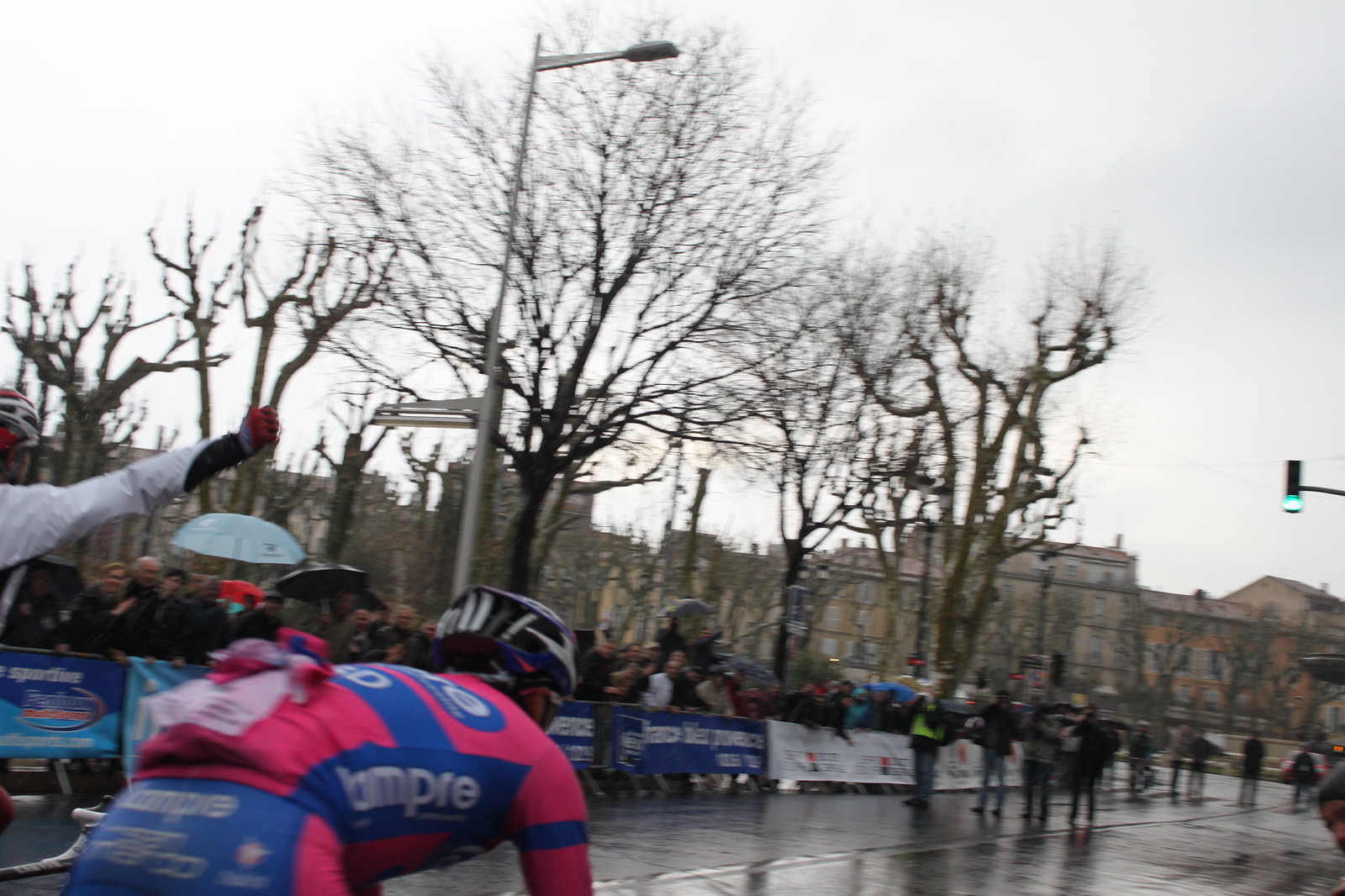The photograph captures a lively bike race set in a big city on a rainy day. The scene is framed with barren trees and urban buildings in the background, contributing to the city's wintry atmosphere. 

In the bottom left corner, a cyclist clad in a form-fitting red and blue outfit, complete with a black and white helmet, is hunched over his bike, focused and heading towards the right side of the frame. Adjacent to him, another cyclist can be spotted raising a red-gloved hand in a victory gesture, though their bike is not visible.

The race course is lined with fences adorned with banners and advertisements, and a large crowd of spectators has gathered behind these barriers. Some bystanders are under umbrellas, suggesting photography enthusiasts with cameras ready to capture the action on the wet road, which is entirely free of cars. A street light can be seen rising among the spectators, and patches of a whitish-blue sky peek through the leafless branches, enhancing the overall brisk and invigorating mood of the event.